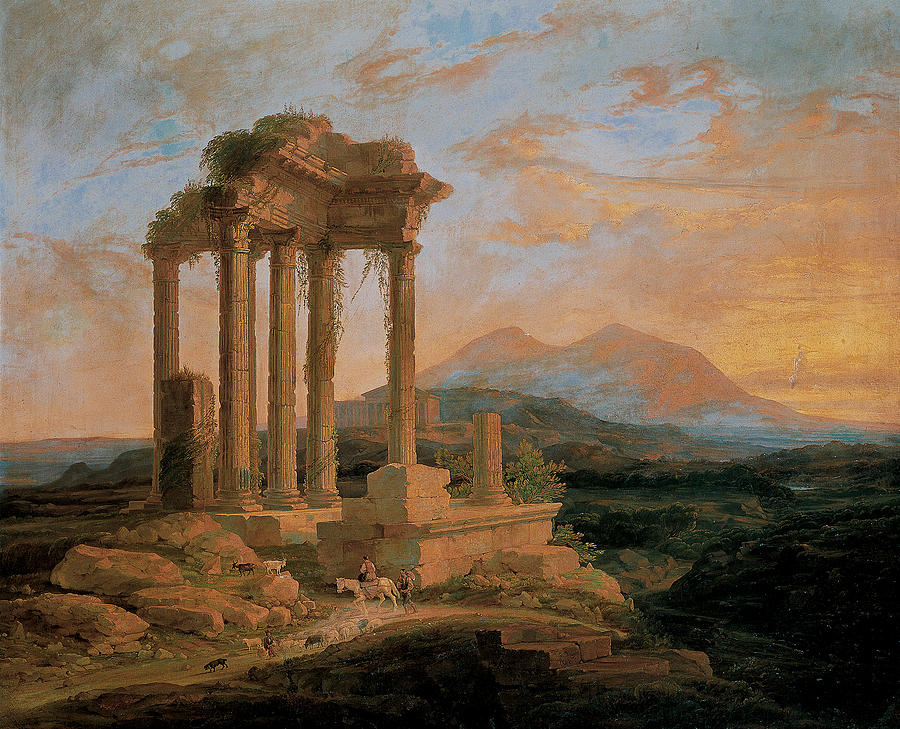This detailed painting features ancient Greco-Roman ruins, specifically a small monument building with six columns, many of which are partially destroyed. The structure, once tall and majestic, now stands in a state of decay. The scene is set against a serene backdrop with a light blue sky adorned with touches of orange and gold, hinting at a setting sun. In the distance, a mountain with an orange-tinted peak rises, adding depth to the composition. Below, rolling green hills and grassy terrain stretch out. In the bottom left of the painting, a shepherd walks alongside a horse carrying a rider, accompanied by a variety of cattle and a dog. This pastoral scene contrasts with the desolation of the ruins, emphasizing the blend of abandonment and life.